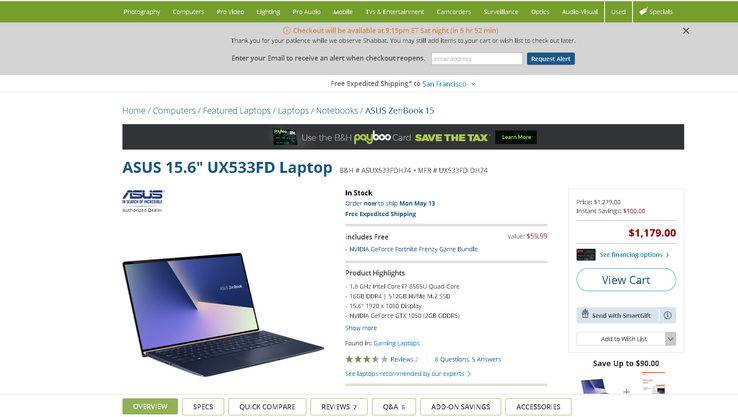The image displays a web page with a structured and layered layout. At the very top, there is a navigation bar featuring multiple text buttons with a white font set against a light green background. Directly beneath the navigation bar is a narrow, gray-background rectangular section containing text. This section also includes a blue button situated in the bottom right corner next to a text field on its left.

Following this section, there is an area with a white background that includes more text. Just below this textual area, a sitemap is presented, showing various links divided by slashes. Further down, there is a prominently placed advertisement, immediately followed by a product page for a laptop.

On the product page, a clear image of the laptop is positioned on the left side. To the right of the image, the price is displayed next to a large "View Cart" button. Centrally located within this section, detailed information about the laptop and available shipping options is provided. At the bottom of the entire web page, several buttons are displayed against a white background. The button on the left side stands out as it is highlighted with a light green color.